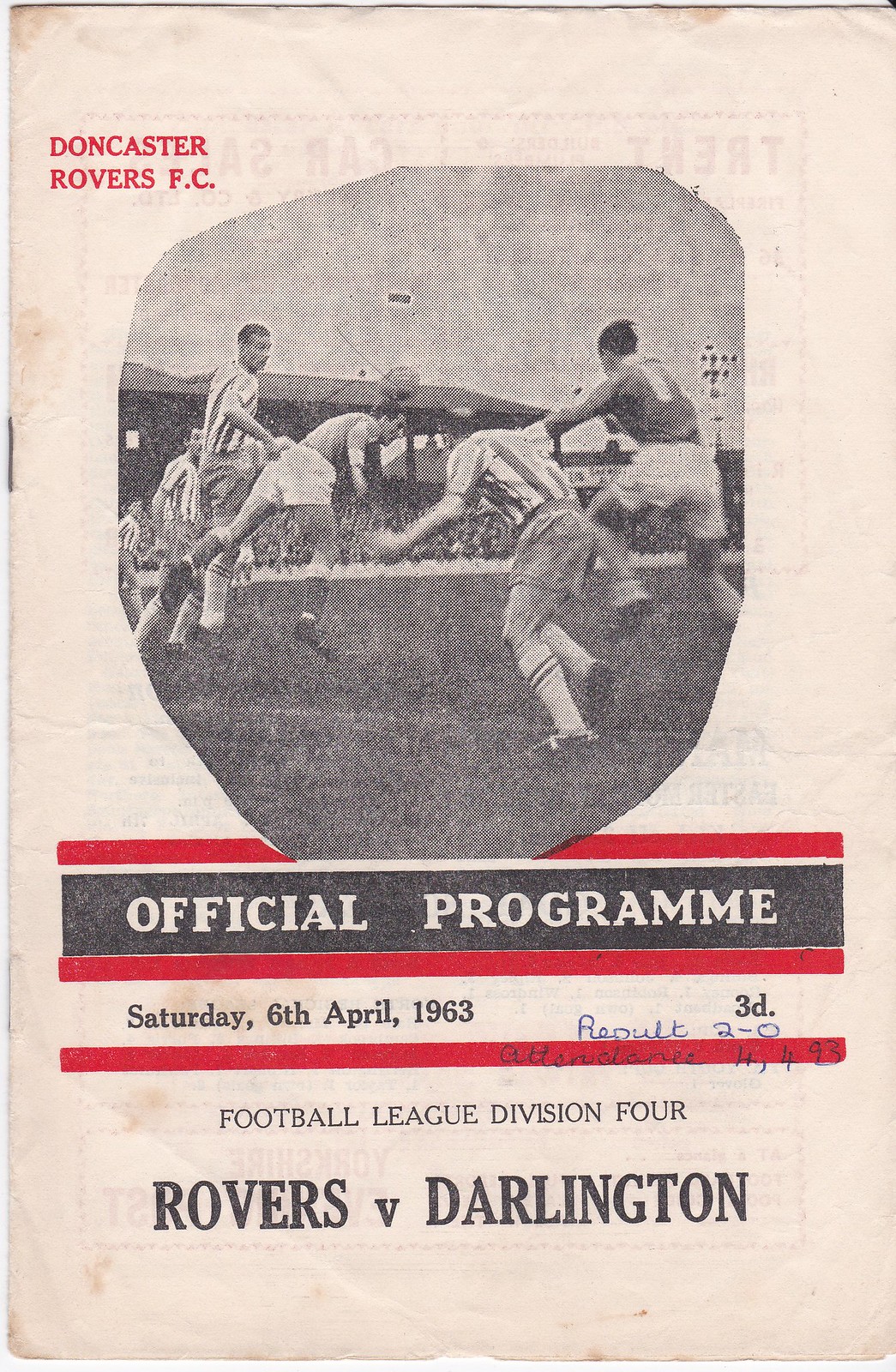This vertical rectangular image portrays an aged, faded poster from the Doncaster Rovers FC. At the top, a black and white photograph of a soccer game, with three officials in striped shirts and three players, one poised to head the ball, is featured. The backdrop includes stands filled with spectators and overhead stadium lights. In the upper left corner, bold red text reads "Doncaster Rovers FC," directly followed by "Official Program" within a black rectangle, flanked above and below by red bars that are partially obscured by the photograph. The date "Saturday, 6th April 1963" is prominently displayed below, alongside handwritten notes indicating the game's score (2-0 written as R-E-P-U-L-T) and attendance (4,493). Further down, the text in black announces "Football League Division 4 Rovers vs. Darlington." The overall color scheme combines gray, white, and red, with the white areas showing signs of aging. The poster's nostalgic charm is accentuated by its vintage design and preserved details.